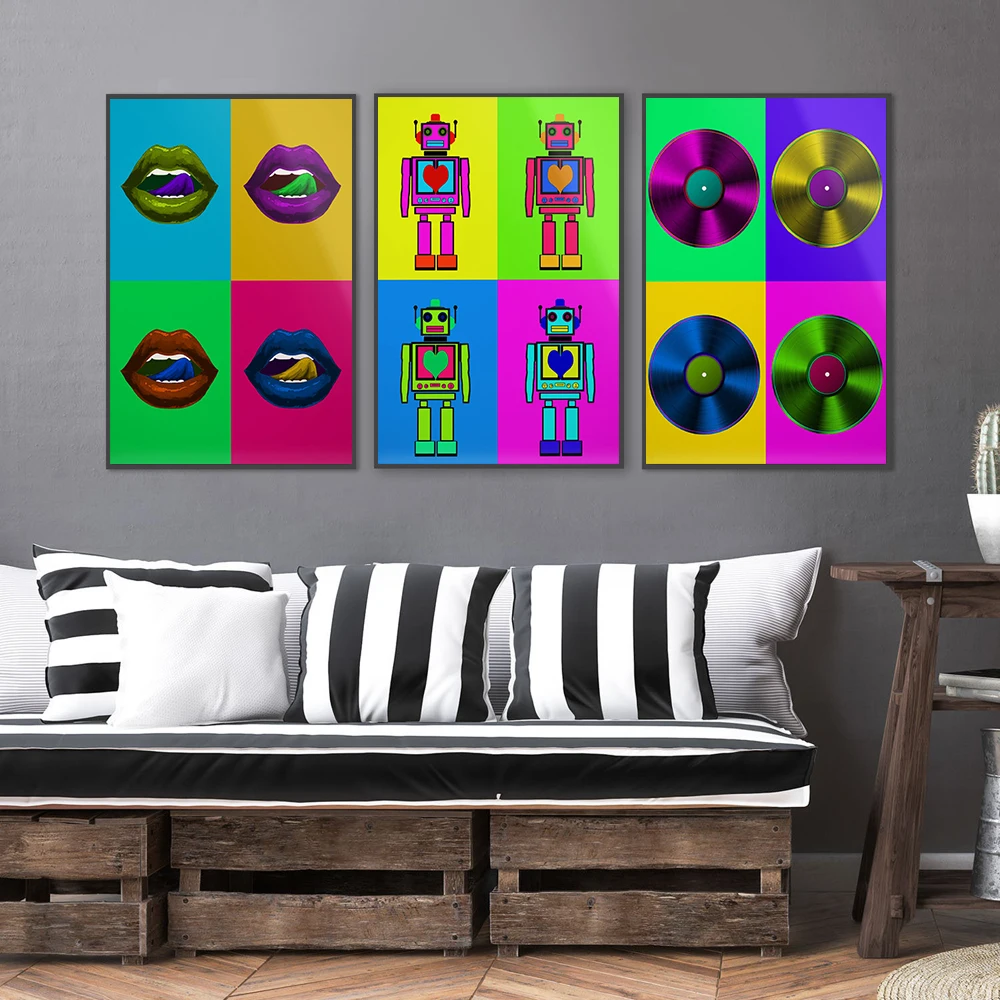The photograph depicts a cozy living room with a hand-crafted wooden couch made from a combination of pallets and wooden crates, featuring black and white striped cushions and pillows. The floor is laid out in a chevron pattern made up of dark, diagonal wooden planks. Against the charcoal-gray wall, three rectangular paintings, each divided into four vibrant sections, are displayed in slim black frames. The left painting illustrates an abstract composition of lips with tongues out, each section boasting a unique color combination. The center painting showcases colorful robots, while the painting on the right features records in various hues. A wooden side table made from the same material as the couch sits to the right, adorned with a white vase containing a cactus. The entire scene is captured in a perfectly square photograph that highlights the vivid, playful art and the rustic, DIY furniture.